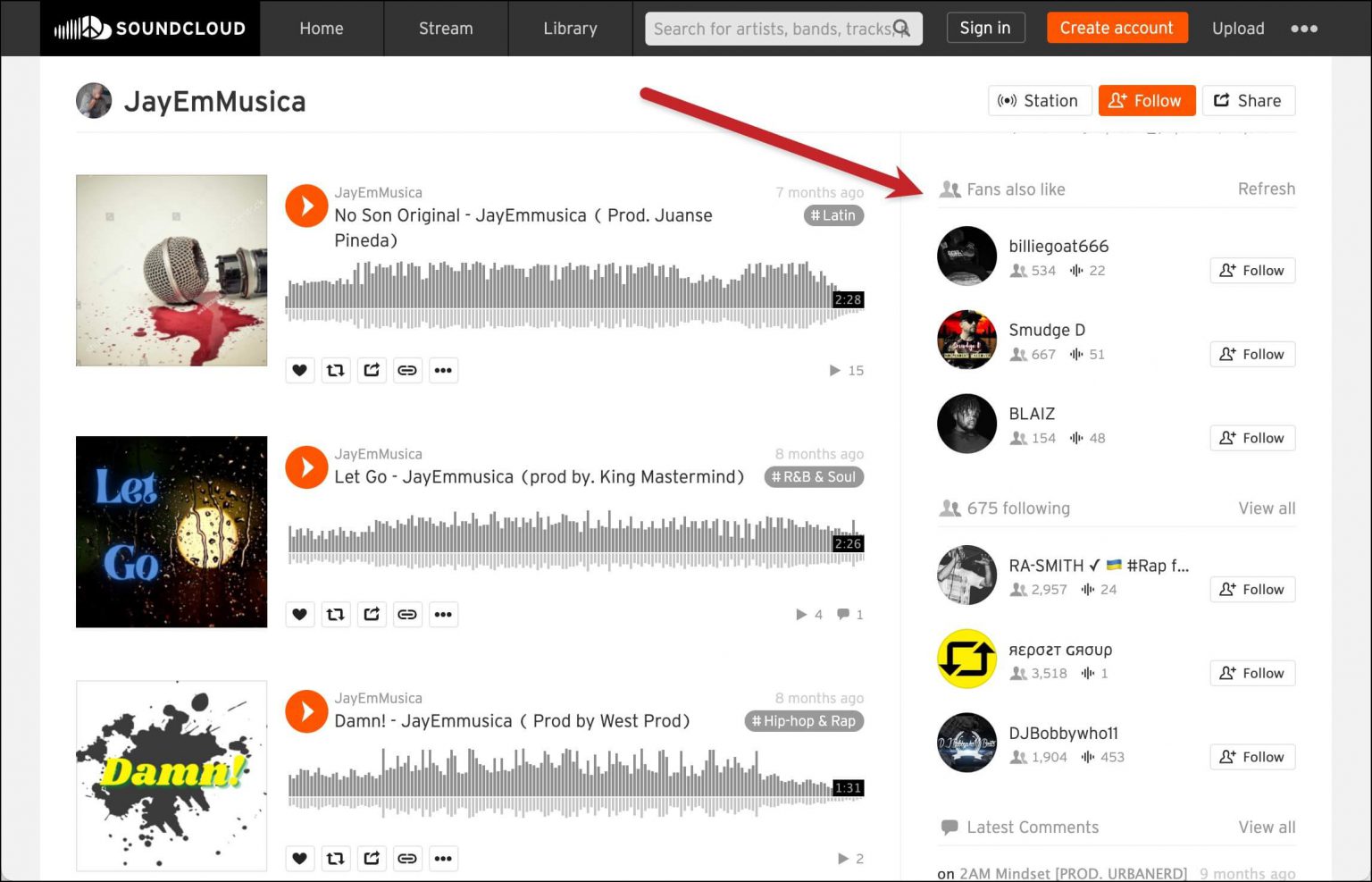The image displays a computer screen featuring a web page layout. At the top, a thin gray navigation bar stretches horizontally across the screen. The leftmost section of this bar is highlighted in black with the white text "SoundCloud." Following this are sequential sections labeled "Home," "Stream," "Library," and a search bar. To the right of the search bar, options for "Sign In," "Create an Account," "Upload," and a menu icon represented by three vertical lines are visible.

On the left side of the image, there is a user profile titled "JM Music." Beneath it, three categories are listed vertically: "No Sun Original," "Let's Go," and "DAM," each accompanied by a small square thumbnail image on their left.

The right side showcases a list of fans and followers. At the top, three follower profiles are listed vertically. Below it, a text indicates "675 following," along with three icons aligned in a row. Each line in this list concludes with a white rectangular button labeled "Follow."